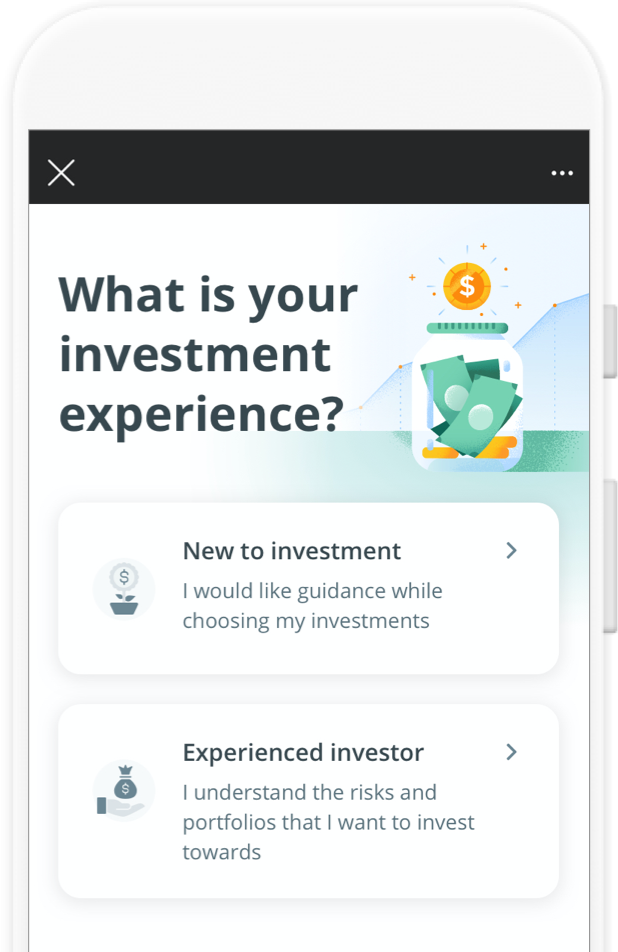The image depicts a screenshot of a mobile phone displaying an investment experience survey interface. The phone, with a sleek white or light gray edge, frames the content neatly. At the top of the phone screen, set against a black bar, is a white 'X' icon on the left and a menu symbolized by three horizontal dots on the right.

Below this bar, the main content area starts with a white background featuring a question in bold black text: "What is your investment experience?" To the right, there is an illustrative graphic depicting a jar filled with green dollar bills and gold coins at the bottom. Above the jar, a yellow circle with a black dollar sign accentuates the money theme. Behind the jar, a blue-toned mountainous landscape adds a scenic touch.

The survey offers two options, each within a white rectangle featuring black text and a small right-pointing arrow icon. The first option reads, "New to investment. I would like guidance while choosing my investments." The second option states, "Experienced investor. I understand the risks and portfolios that I want to invest towards." These selections aim to categorize the user's investment background for tailored guidance.